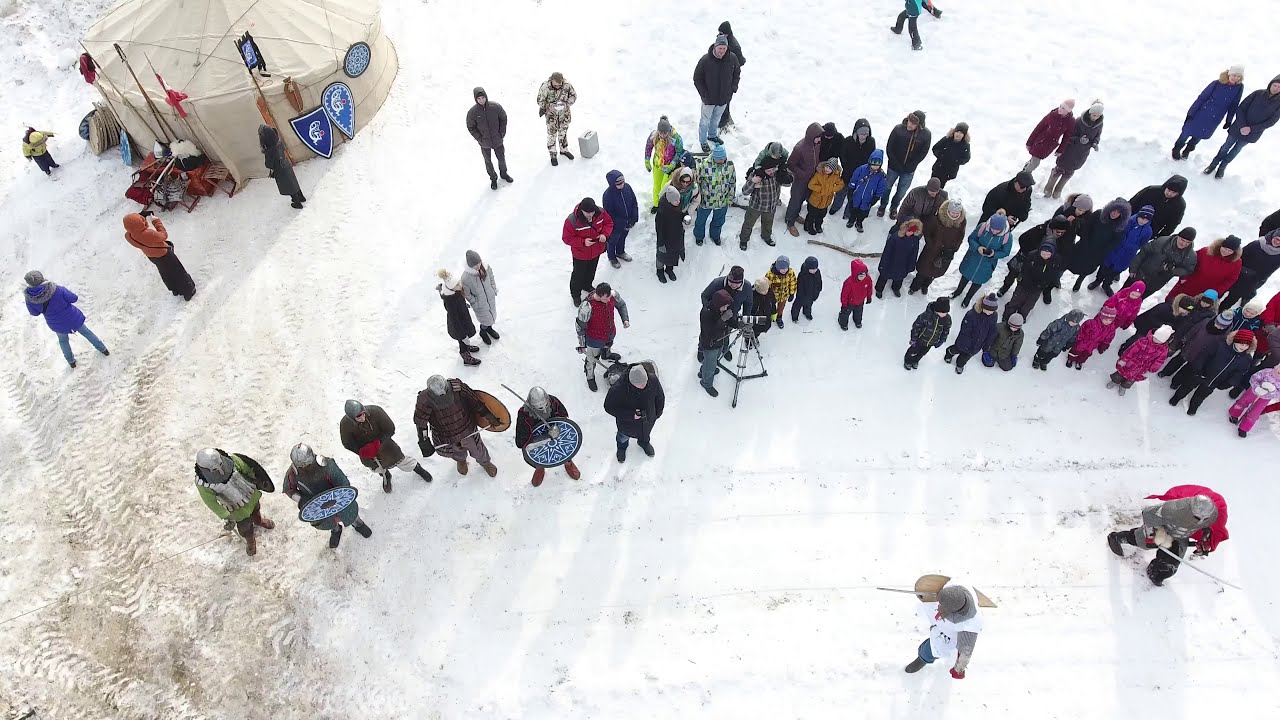The image depicts a bustling scene at what appears to be a medieval-themed event taking place outdoors on a snow-covered ground. In the snowy landscape, a diverse group of around 50 people, ranging from children to adults, are bundled up in heavy coats and snow pants against the cold. Many individuals are dressed in medieval attire, sporting chain mail, headgear, and wielding swords and shields. In the top left corner, a roundish off-white tent adorned with shields and symbols serves as an apparent staging area for the participants, complete with stands and a bench holding equipment. The snow underfoot shows signs of activity, with dirty brown patches and footprints suggesting recent motion and preparation, perhaps even plow tracks clearing space for the event. Spectators, who are mostly children, gather around, seemingly focused in one direction as they await what might be a jousting or sword-fighting demonstration. At the center of the scene, someone is prominently filming the event with a camera on a tripod, capturing the lively atmosphere and medieval reenactment amid the wintery setting.